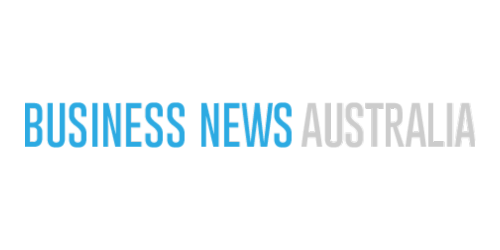A stark, minimalist design featuring a clean, white background is punctuated only by a single line of text. In a tight, sans serif font, the words "BUSINESS" and "NEWS" appear in a striking royal blue, while "AUSTRALIA" is rendered in a muted gray. All text is capitalized, emphasizing a no-nonsense approach, with reduced kerning giving the words a compact and structured appearance. The simplicity of the image draws focus entirely to the text, suggesting a straightforward, perhaps austere presentation of information.